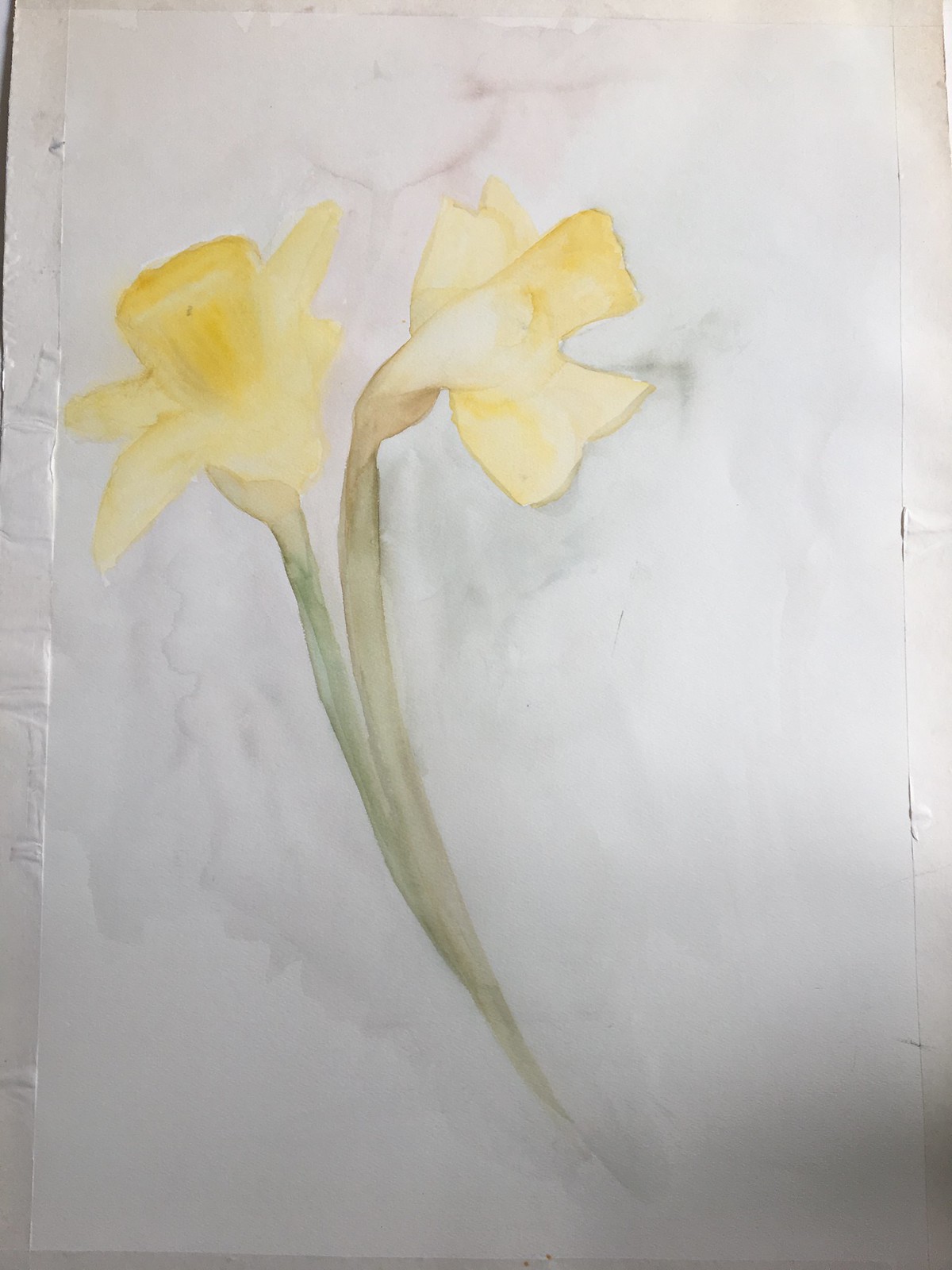This is a detailed photograph of a watercolor painting, prominently featuring two yellow flowers, likely daffodils, on a tall rectangular canvas or thick piece of paper. The flowers, painted in light yellow with darker yellow centers, have fluid and loose petals that give a delicate and soft appearance. The green stems, which fade to a lighter green and brown near the base, appear flabby and non-rigid, extending downwards almost disappearing at the bottom of the canvas. The painting includes subtle background details with grey and green tinting around the flowers and a faint touch of pink above them to add depth. Some black markings and water stains are visible, indicating that water has pooled on the canvas, further emphasizing its watercolor medium. The canvas sits on a white surface, possibly a table or desk, and there are vertical tears on the edges, giving the paper an off-white and slightly torn appearance. The composition provides a gentle, almost ethereal quality to the artwork, focusing on the fragile beauty of the flowers.